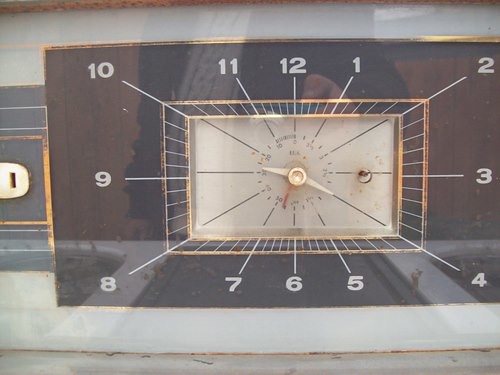A close-up photograph captures the intricate details of a vintage, rectangular-shaped clock. The clock features multiple layered rectangular designs. At the center, a white rectangular face is adorned with intersecting lines converging at the hands of the clock. The minute hand points at the four, while the hour hand rests just past the nine, indicating a time of 9:20. Beyond the white face, a gold rectangular pattern with fine lines encircles it. This pattern is bordered by another gold rectangle, which frames a blackish-gray backdrop. Surrounding the clock face, the numerals 1 through 12 are clearly visible, completing the elegant and nostalgic design of the timepiece.